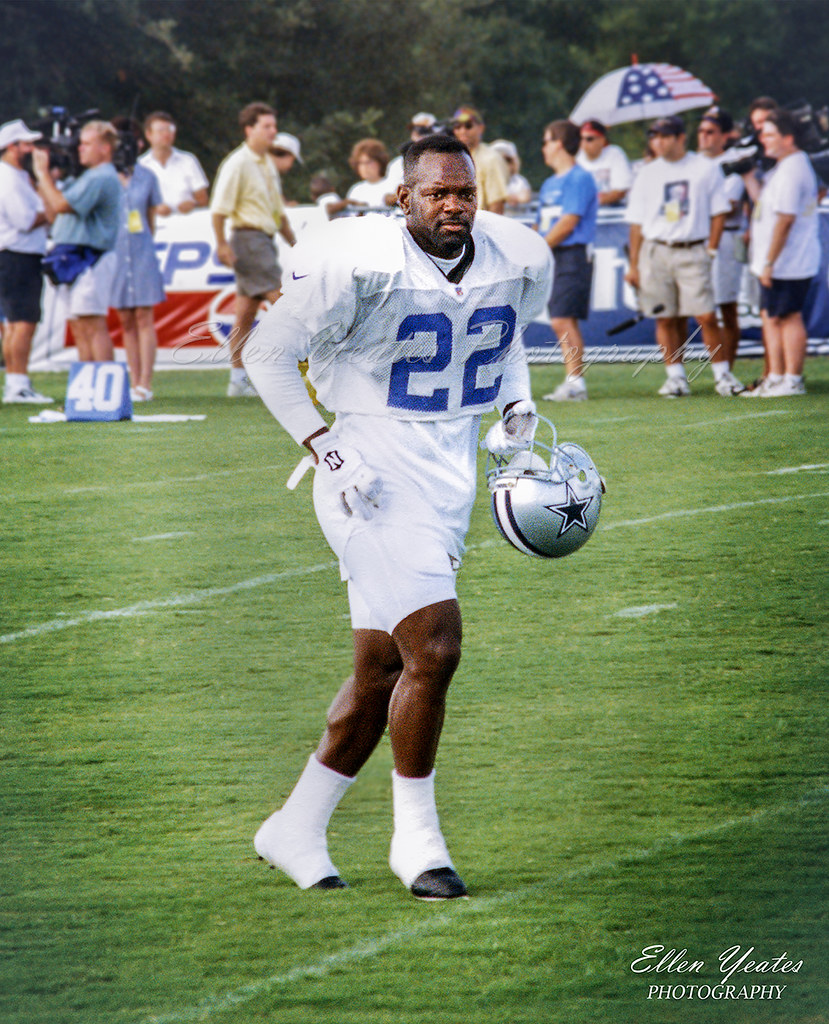This professional-quality photograph, taken by Ellen Yeats Photography, captures a Dallas Cowboys football player walking on a green football field marked with white lines. The player, wearing a white jersey and shorts with the blue number 22 prominently displayed on his chest, carries a silver helmet emblazoned with the team’s iconic navy blue five-sided star outlined in white. He is outfitted with white socks, white shoes, and white gloves marked with an 'N'. 

The player, who has dark skin, short dark hair, and a slight mustache or beard, is positioned at the center of the image with numerous spectators and photographers visible in the background. Among them, a man in a blue top holds a large video camera, and others in yellow and blue shirts are gathered around. The scene also includes several umbrellas, one designed like an American flag, and a visible Pepsi advertisement logo. Additionally, a small yard marker with the white number 40 on a blue background is placed on the field. The photograph's bottom right corner features the photographer's name, Ellen Yeats, in flowing script followed by "PHOTOGRAPHY" in all capital letters.